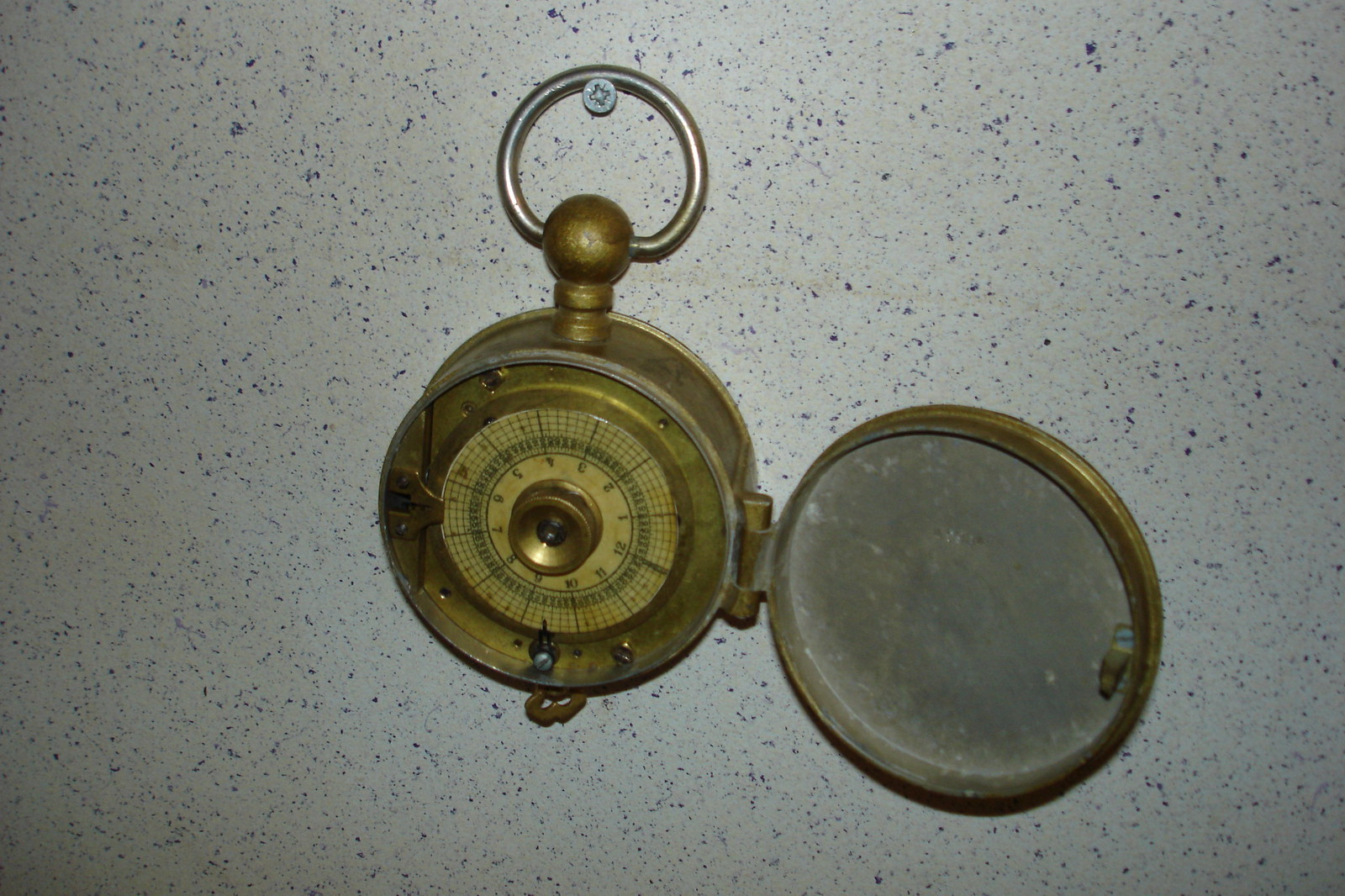This image features a vintage gold pocket watch, characterized by its circular shape and antique appearance. The golden structure, likely made of brass, is small enough to fit comfortably in a pocket. At the top, there is an oval-shaped hook, leaning more towards a circular design, which attaches to a bulbous, ornate piece typically used to secure the watch on a chain or fob.

The watch face is inscribed with numbers ranging from 1 to 12, much like a traditional clock. However, the watch's hands are missing, rendering it non-functional for telling time. The absence of the hands suggests the watch may have been damaged over time, which aligns with its overall vintage look.

The outer case of the watch is open, showcasing the internal hinge mechanism and the brassy front cover that would normally snap shut to protect the watch face. The watch is currently suspended from a screw, which is embedded into a speckled wall, giving the impression that it is on display in this peculiar manner.